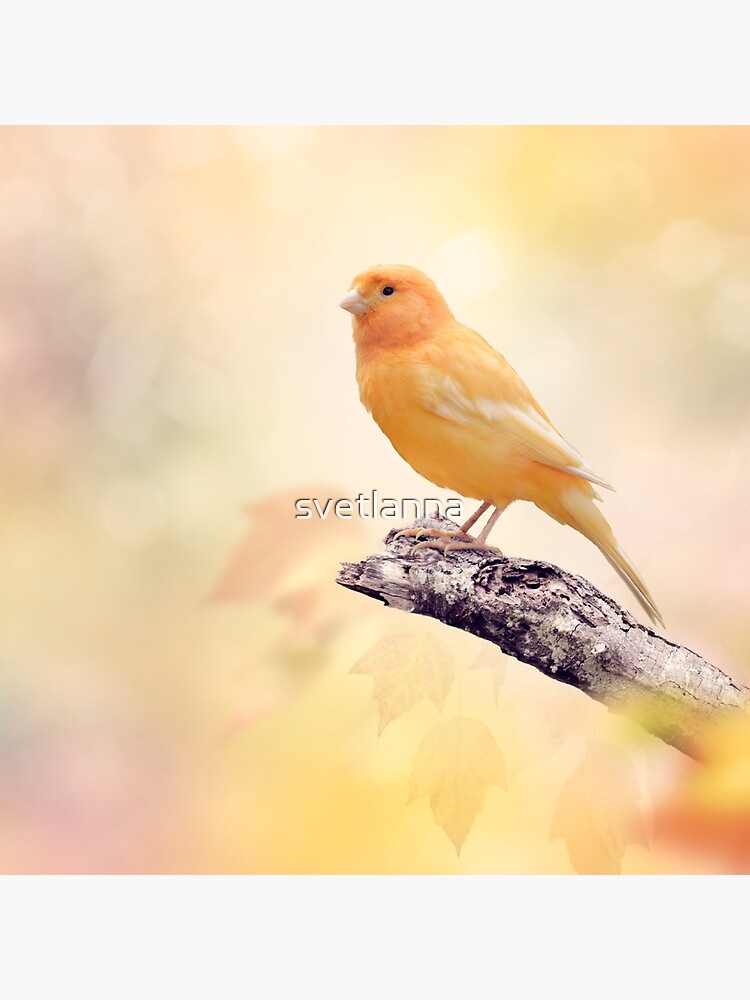The image appears to be a highly detailed photo, possibly mistakable for a hyper-realistic painting due to its meticulous rendering. The focal point is a small bird, which resembles a chickadee but has unique coloration: a light beak, black eyes, a vibrant tangerine-colored head, and lighter orange and white hues throughout its body. The bird is depicted perched on a piece of tree bark at the end of a bare branch. The branch itself is a mix of black, white, gray, and brown shades, adorned with subtle traces of green.

This branch extends into the bottom right of the image, while the bird is centered slightly off to the right. Behind the bird, the background blurs into a radiant, almost ethereal mix of colors, including white, pink, red, green, gold, yellow, and orange. This blurred foliage effect creates a luminous, glowing ambiance. Notably, the name "Svetlana," written in white, appears in the middle of the image. While the bird and branch are in sharp focus, the background provides a soft, colorful glow that enhances the overall sense of light and warmth.